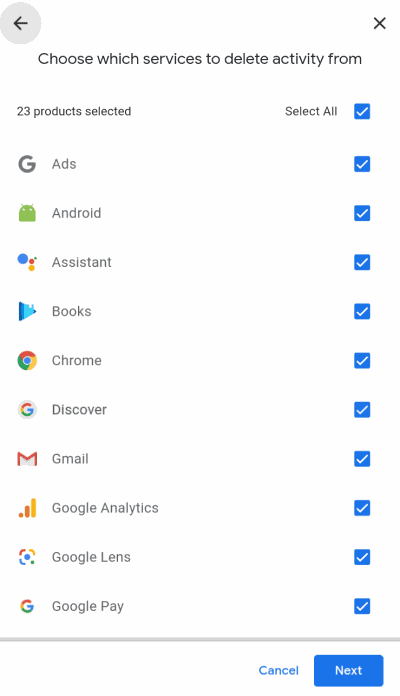This screenshot captures the settings screen of a mobile app, designed to manage activity deletion from various services. At the top of the screen, there's a navigation element featuring a gray circle with a left-pointing arrow, and a "X" on its right. Centrally aligned beneath this, the header text reads "Choose which services to delete activity from."

Below the header, there's an indication of selection, stating "23 products selected" on the left, and an option to "Select All" on the right. The layout is organized with app names listed down the left side and corresponding checkboxes down the right side, all of which are selected.

Prominent app names include Google Ads, Android Assistant, Books, Chrome, Discover, Gmail, Google Analytics, Google Lens, and Google Play. The background of the screen is white, providing a clean and clear backdrop for the content.

At the bottom of the screen, a horizontal gray bar delineates the app list from the action buttons. Positioned at the bottom right, there's a "Cancel" button, followed by a blue "Next" button to its right, facilitating navigation through the settings options.